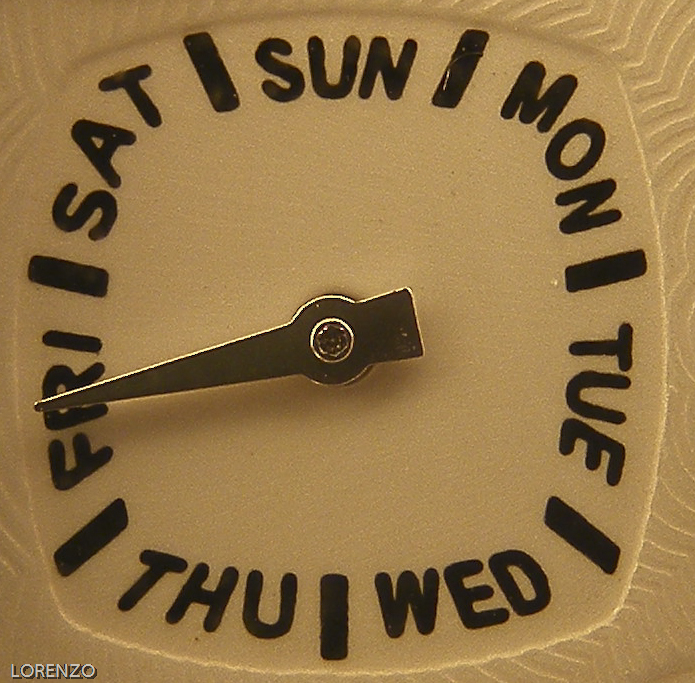This image showcases a close-up of a unique weekly calendar dial, which appears to be made of either ceramic or wood. The dial is square-shaped with a rounded appearance and a light golden brown or cream background. The edges are indented with subtle lines, reminiscent of the edge of a plate, and the overall texture suggests a hand-painted finish. In the bottom left corner, the name "Lorenzo" is prominently displayed in white, capital letters.

The calendar features the days of the week written in large, dark brown or black letters, arranged in a circular format around the face of the dial. Starting from the top center and moving clockwise, the days are abbreviated as SUN for Sunday, MON for Monday, TUE for Tuesday, WED for Wednesday, THU for Thursday, FRI for Friday, and SAT for Saturday. A single golden metallic arrow hand is positioned to indicate the current day, which in this image, is pointing to Friday.